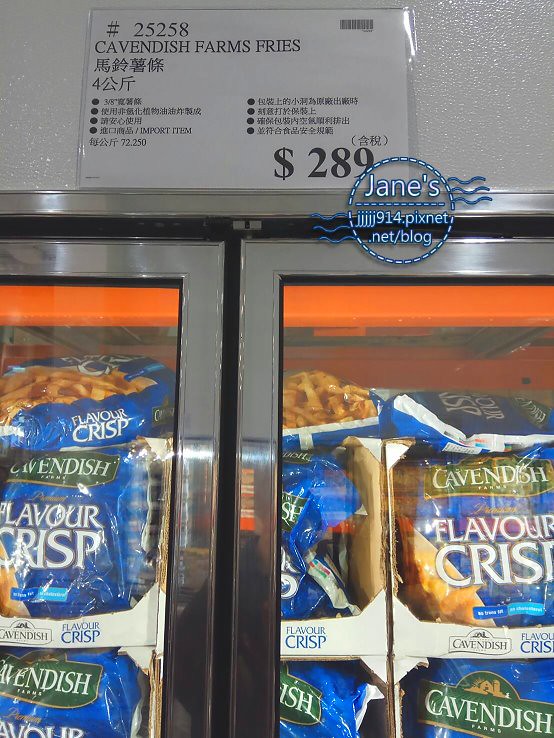This portrait-mode image, likely taken at a grocery store such as Costco, captures the top section of a refrigerated unit indoors. Prominently displayed above the freezer doors is a laminated white sign marked with "25258 Cavendish Farms Fries" in black print, followed by Asian characters detailing the product. In the lower right corner of the sign, the price $289 is displayed. Overlaying this scene is a blue circled watermark with the text "Jane's jjjj914.pixnet.net".

Below the sign, the refrigerator unit is partly obscured by its clear glass doors, but inside, it is filled with boxes containing blue bags of Cavendish Flavor Crisp fries. The bags feature white lettering and a green Cavendish Farms logo, with enticing images of golden crisps visible on the packaging. The arrangement of the boxes suggests they are stored in the same cardboard boxes in which they were shipped.